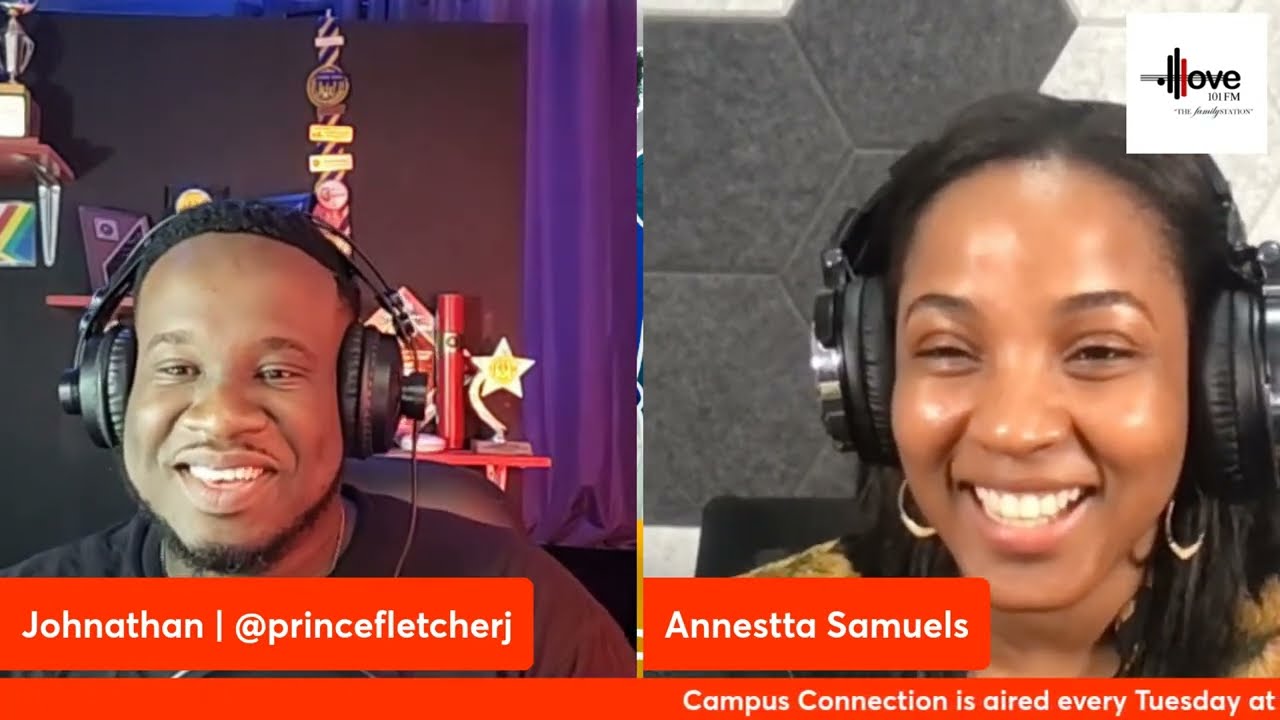The screenshot from a video chat features two smiling individuals, both wearing large black headphones. On the left is Jonathan, identified by his caption "Jonathan @ Prince Fletcher J" in white text on an orange background. Behind him are trophies on a shelf, suggesting a personal or professional achievement display. On the right side is a woman named Anesta Samuels, indicated by her name in white text within a red square below her image. Anesta is wearing earrings and a yellow shirt, positioned in front of a background featuring hexagonal gray tiles. At the bottom of the image, white text on a red background reads "Campus Connection is aired every Tuesday at". A logo at the top right of the image indicates the radio station "Love 101 FM Family Station". Both Jonathan and Anesta appear to be enjoying a lively conversation, signified by their bright, genuine smiles. Jonathan is dressed in a black shirt, suggesting a casual yet polished appearance fitting for a radio or virtual event.